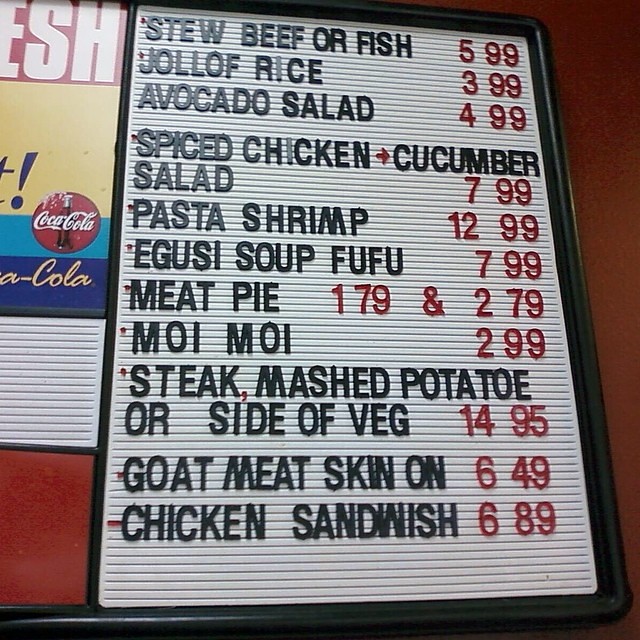The image showcases a retro-style, fully analog menu board at a restaurant. The board features a white background with hand-placed individual black plastic letters, displaying a variety of dishes and their prices. The menu, described from top to bottom, starts with "Stew Beef or Fish" priced at $5.99, followed by "Jollof Rice" for $3.99. Next is "Avocado Salad" for $4.99 and "Spiced Chicken" leading to "Cucumber Salad" at $7.99, indicated by a red arrow.

Further down the menu, "Pasta Shrimp" is listed for $12.99, followed by "Goosey Soup Fufu" at $7.99. "Meat Pie" is offered at two prices, $1.79 and $2.79, likely for different sizes. "Moi Moi" is next, priced at $2.99, and "Steak Mashed Potato or Side Veggie" follows at $14.95. "Goat Meat Skin" is listed for $6.49, and "Chicken Sandwich" (misspelled as 'Sand Wish') is priced at $6.89.

All text is displayed in dark red, matching the deep red background of the board. To the left, the edge of a Coca-Cola poster is partially visible, adding a touch of branded decor to the vintage setup.